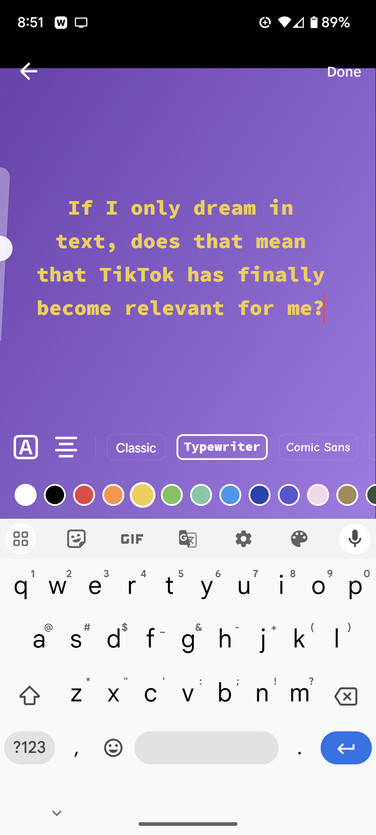This descriptive caption captures the nuances of the image:

"A screenshot of a cell phone displaying an Instagram post in progress. The screen features a purple background with gold text centered that reads, 'If I only dream in text, does that mean that TikTok has finally become relevant for me?' Below the text, a horizontal array of color options is shown, allowing the user to change the background color. Above these color options, an icon with an 'A' in the center suggests font customization options like 'classic,' 'typewriter,' and 'comic sans.' The bottom section of the screen displays the phone's keyboard pop-up, featuring various icons for emojis, inserting photos, GIFs, painting, and using a microphone. The QWERTY keyboard is also visible, with specific keys: a gray button for numbers and symbols ('?123') on the bottom left, followed by a comma key, a smiley face icon, the space bar in the center, and the return/send button in blue on the bottom right."